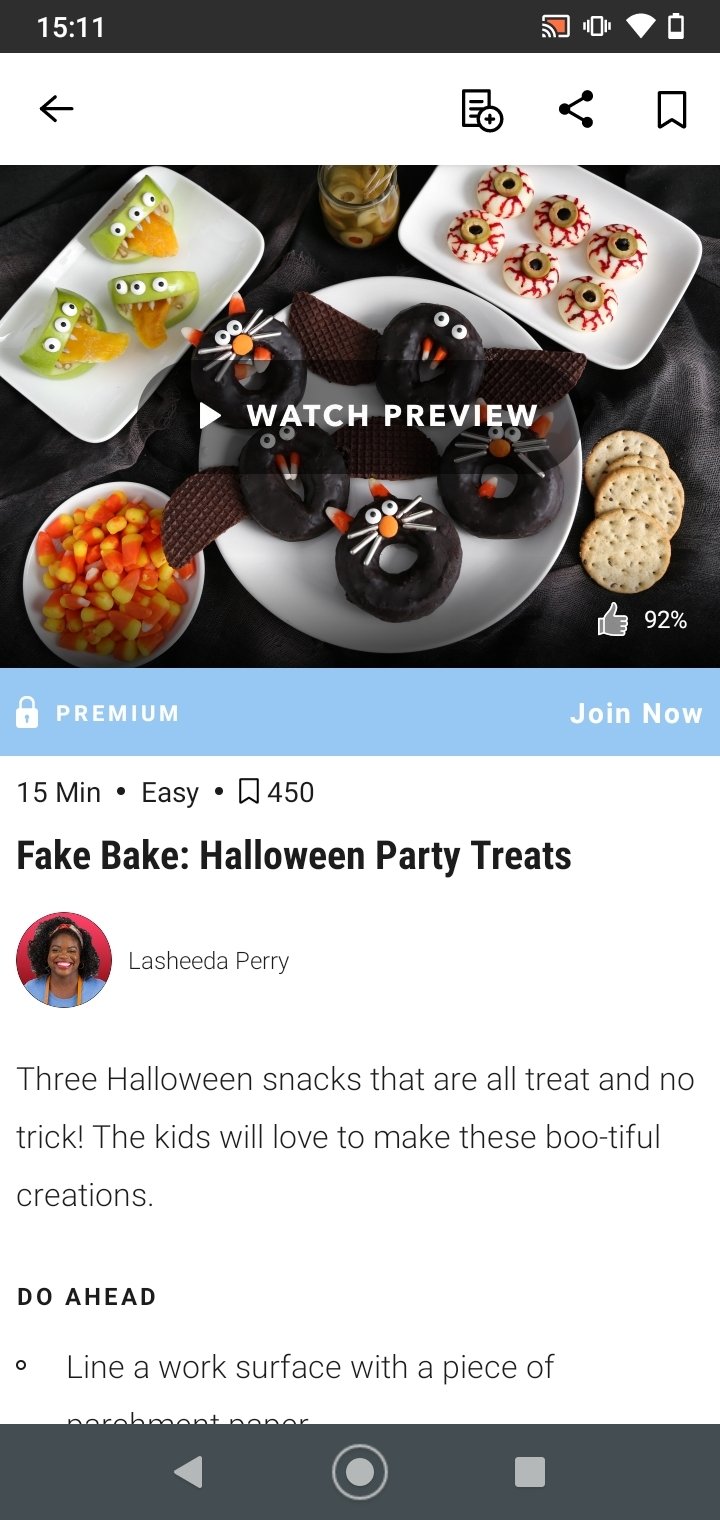Lashita Perry introduces a collection of creative and fun Halloween treats in a detailed video tutorial designed for families to enjoy together. The video is accompanied by a pre-order option—joining now grants access to the full content. The segment emphasizes how easy these treats are to make, with a preparation time of just 15 minutes. An impressive 450 users have bookmarked this tutorial, and it holds a high approval rating with 92% of viewers liking the video.

The title, "Fake Bake Halloween Party Treats by Lashita Perry," is complemented by a cheerful image of Perry herself. The tutorial highlights three Halloween snacks—playfully described as "all treat, no trick." These delightful creations are guaranteed to be a hit with kids. The instructions start with a tip: line your work surface with parchment paper.

The visual examples include various themed plates of food. The centerpiece features a black-frosted donut designed to resemble a black cat, complete with candy corn ears and nose, icing whiskers, and candy eyes. Other treats showcased include saltine crackers styled for the occasion and green monster-themed snacks with three eyes and tongues sticking out.

Embedded in a sleek black bar at the top of the video are the current time (15:11), Wi-Fi status, and screencasting indicators. The option to join the premium subscription is displayed against a blue border in white text. This engaging content not only promises a fun culinary experience but also provides clear, easy-to-follow instructions, making it perfect for family Halloween celebrations.